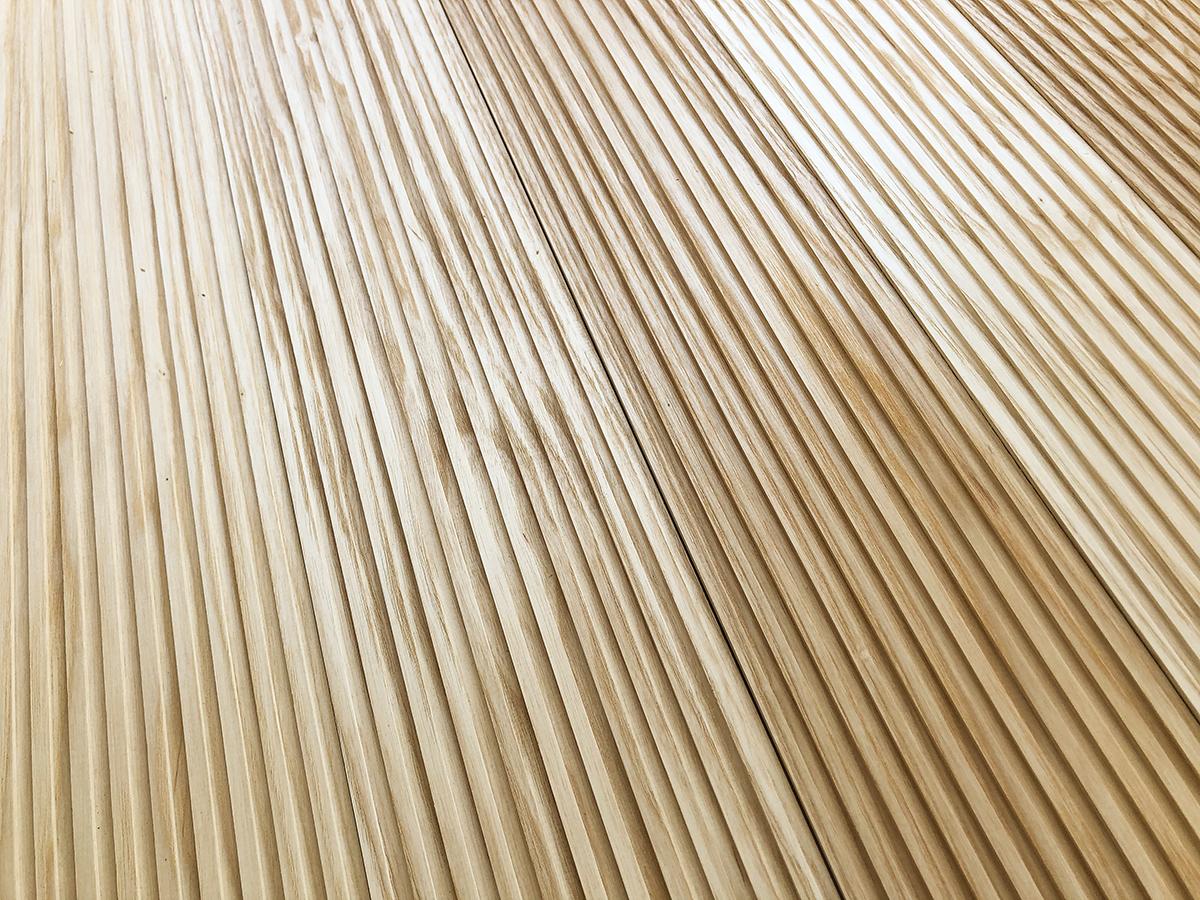The image depicts a well-lit close-up of a tan and brown wooden surface, most likely floor paneling or wall paneling. The surface features numerous vertical lines or strands, predominantly cream-colored with occasional darker brown streaks, giving it a striped, textured appearance. The lines appear parallel and finely carved, suggesting machine craftsmanship. The photograph is angled slightly, emphasizing the vertical direction of the wood grains and grooves, which vary slightly in color across the surface. The light hits the surface from the right, highlighting the natural wood grain and ridges, although the exact context of the paneling within a larger structure remains unclear.